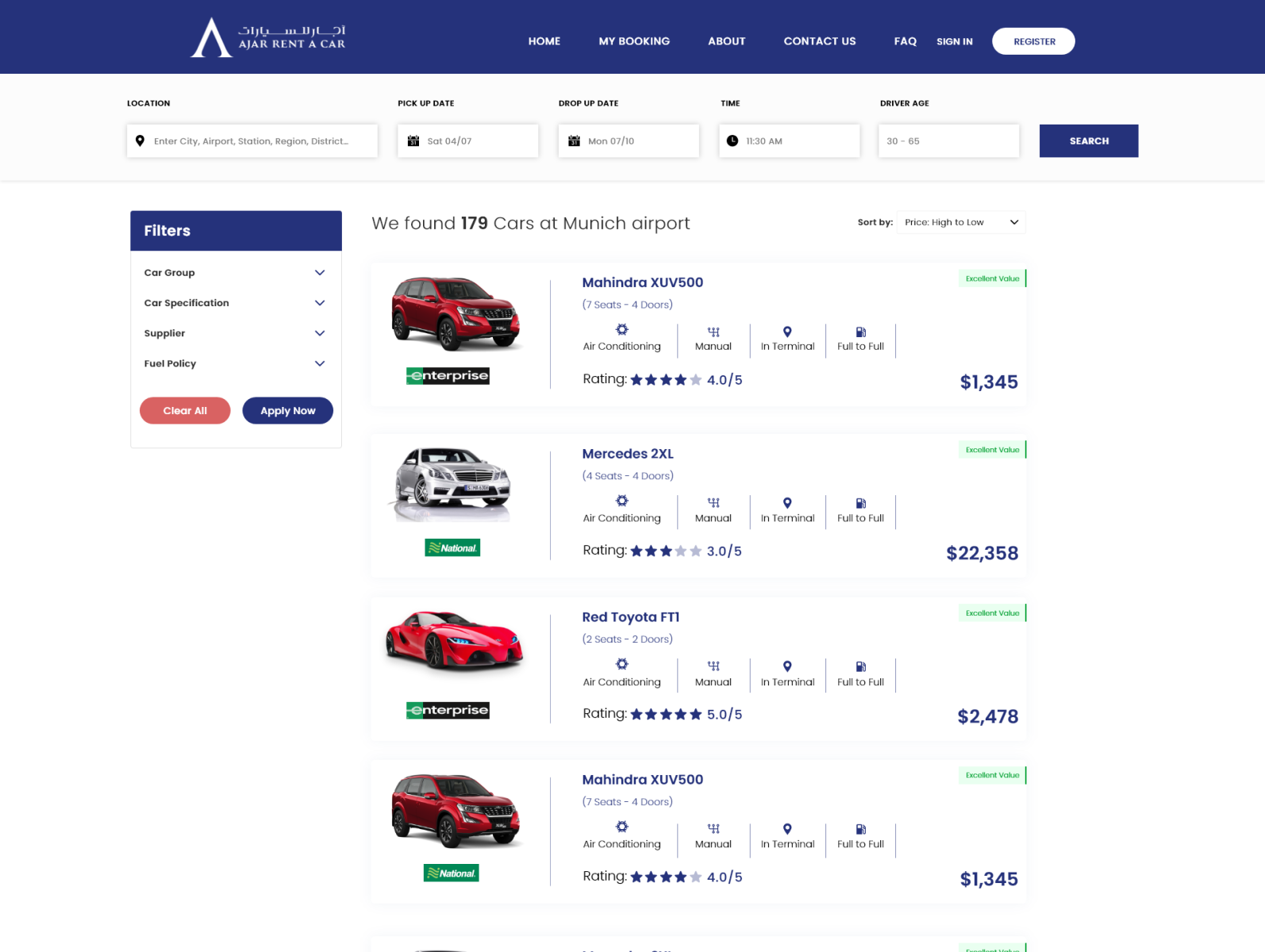The webpage for a car rental service is dominated by a royal blue horizontal banner at the top, stretching from left to right. On the left side of this banner, slightly more than a quarter of the way from the edge, sits the logo—a white, sans-serif letter resembling an uppercase 'A' but missing the horizontal bar.

To the right of the logo, the banner features various navigation headings in bold, capitalized white font: HOME, MY BOOKING, ABOUT, CONTACT US, FAQ, and SIGN IN. A white oval button with the word 'REGISTER' in navy font is also present.

Beneath the banner, the page is organized into different sections. The central section houses search functionalities in horizontal input boxes, each labeled with bold, capitalized, black font. These boxes are designated for LOCATION, PICKUP DATE, DROP-OFF DATE, TIME, and DRIVER (text unclear). A blue search button with 'SEARCH' in white letters lies adjacent to these input boxes. 

To the left, a vertical rectangular sidebar with a white background offers filtering options. The sidebar includes menus for car group, car specification, supplier, and fuel policy, each marked by a small blue down-pointing arrow. At the bottom of this sidebar, two horizontal buttons allow users to clear selections or apply filters: one coral-colored with 'CLEAR ALL' in white font, and the other blue with 'APPLY NOW' in white font.

In the main content area to the left of the center of the page, there is a summary in black font: "We found 179 cars at Munich airport," where '179' is in bold font. 

Four listings of available cars are displayed in a vertical column. Each listing includes a picture of the car on the left. The first and third listings have a rectangular bar below the image with "Enterprise" labeled in black and green. The second and fourth listings feature a similar green bar, likely labeled "National" in white font, though it is unclear. 

Details for the first car, a Mahindra, include unreadable specifications except for air conditioning and a 4.0 out of 5 rating shown via four blue stars, priced at $1,345. The second car, a Mercedes XXL, has similarly unreadable details, a rating of 3.0 out of 5 stars with three blue stars, and is priced at $22,358. The third car, a red Toyota FTI, carries a perfect rating of 5.0 out of 5 stars, priced at $2,478. The fourth car, another Mahindra, has a 4.0 out of 5 rating shown by four blue stars and is priced at $1,345. Each listing appears to include additional green text, but it is too small to discern.